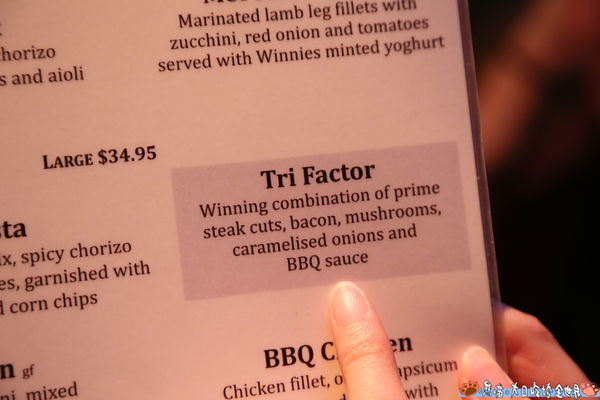In this close-up image taken at a restaurant, the primary focus is on a menu with a white, laminated background, indicating wear on the edges. Central to the image is a right-hand finger pointing to a highlighted menu item in a gray box. The featured dish, labeled "Trifactor," is described in bold black letters as a "winning combination of prime steak cuts, bacon, mushrooms, caramelized onions, and barbecue sauce." Above this selection, the menu details a dish of "marinated lamb leg fillets with zucchini, red onion, and tomatoes served with Winnie's minted yogurt" and a price marked as "large $34.95." Surrounding the main item, only bits of other menu items are visible, including "spicy chorizo garnished with corn chips" to the left, and a partially obscured "barbecue chicken" and "chicken fillet" below. A small, difficult-to-read logo with blue and brown hues is tucked away in the lower right corner of the image.